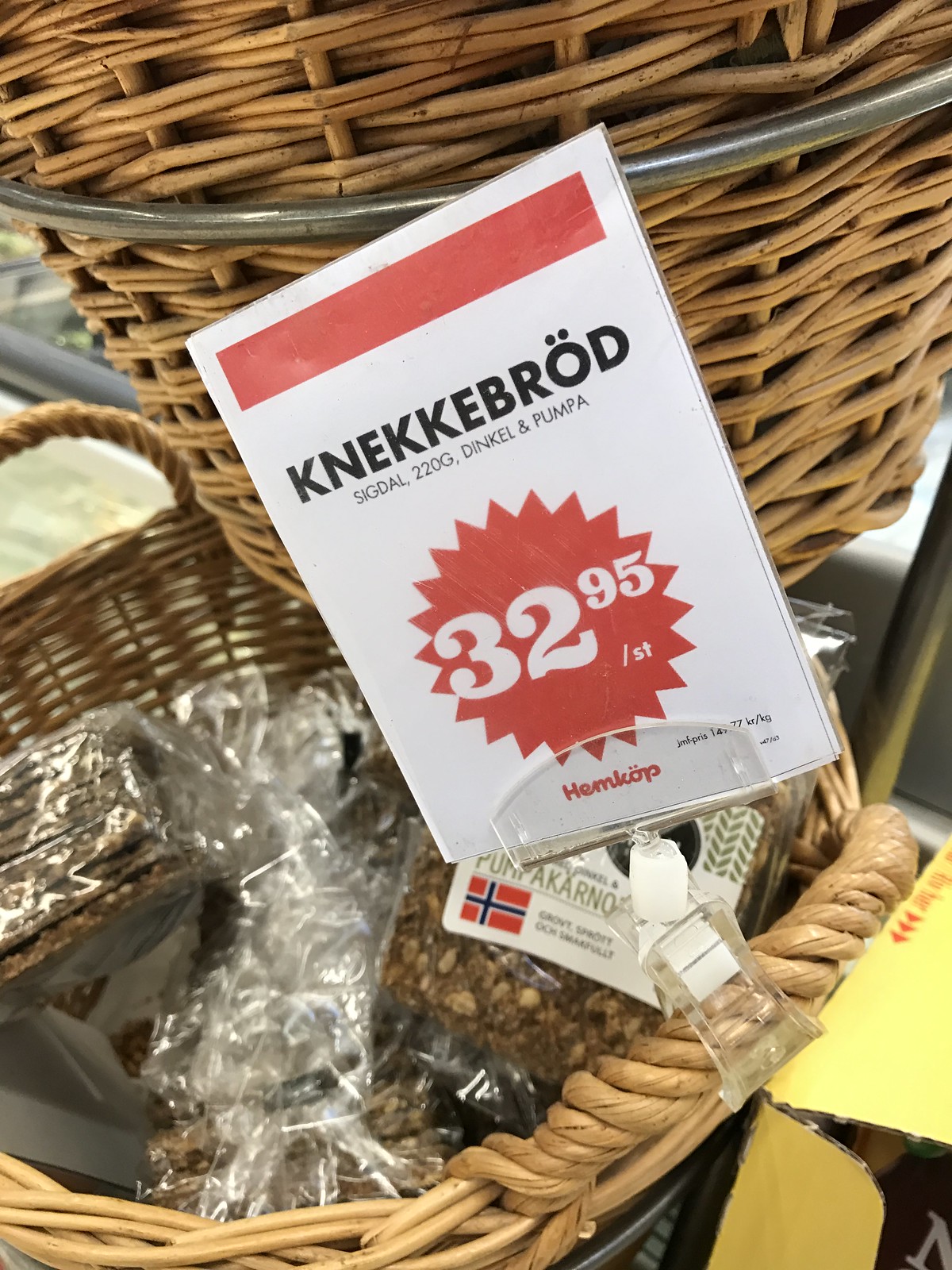The image captures a scene inside a grocery store or market, focusing on a display rack made of metal framing that holds woven wicker baskets stacked one atop the other. The photo zooms into the lower basket, which contains cellophane-wrapped packages of what appear to be food items that resemble flat, brown granola bars or possibly seeds. Attached to the basket is a plastic clip holding a rectangular white tag. The tag, adorned with a red bar at the top and a red starburst effect, has text in a foreign language that appears to be Dutch, saying "Knekkerbrød Broadsig Doll 20 220g Dinkel og Pumpernickel". The price is prominently displayed as $32.95 per item. Additionally, the tag features a red flag with a blue cross, indicating the product's country of origin. The brand name visible on the tag is Hemcorp.